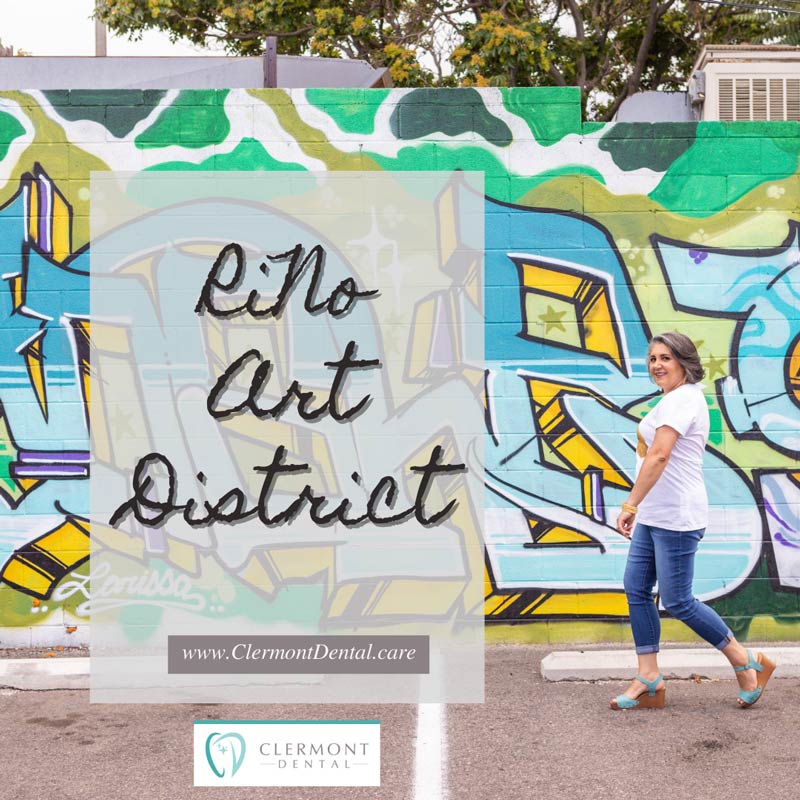The image is a detailed advertisement for Claremont Dental, prominently showcasing their branding and contact information against a visually striking backdrop. The scene captures a woman walking across an asphalt parking lot, marked by a white line and flanked by smooth concrete parking bumpers. The centerpiece is a large brick wall adorned with a vibrant graffiti mural in shades of blue, green, white, and dark yellow. The mural features illegible blue and yellow-outlined text, with a signature "Larissa" visible in the bottom left corner. Above the wall, a few trees can be seen.

The woman in the photograph, an older lady with short gray hair, is dressed in a white t-shirt, blue capri jeans, and brown tall clogs with blue straps. She is positioned on the right side of the frame, walking and looking at the camera with a smile.

Overlaying the photograph is a white translucent text box situated along the left side of the frame. This box contains bold black script reading "Rino Art District," with "Rino" stylized as "Re-Know" (capital R, lowercase i, capital N, lowercase o). Beneath this, a smaller dark gray box with white text features the URL "www.claremontdental.care". At the bottom, a white rectangle with a blue line on top and a blue swirl logo to the left side complements the Claremont Dental name in gray text on the right.